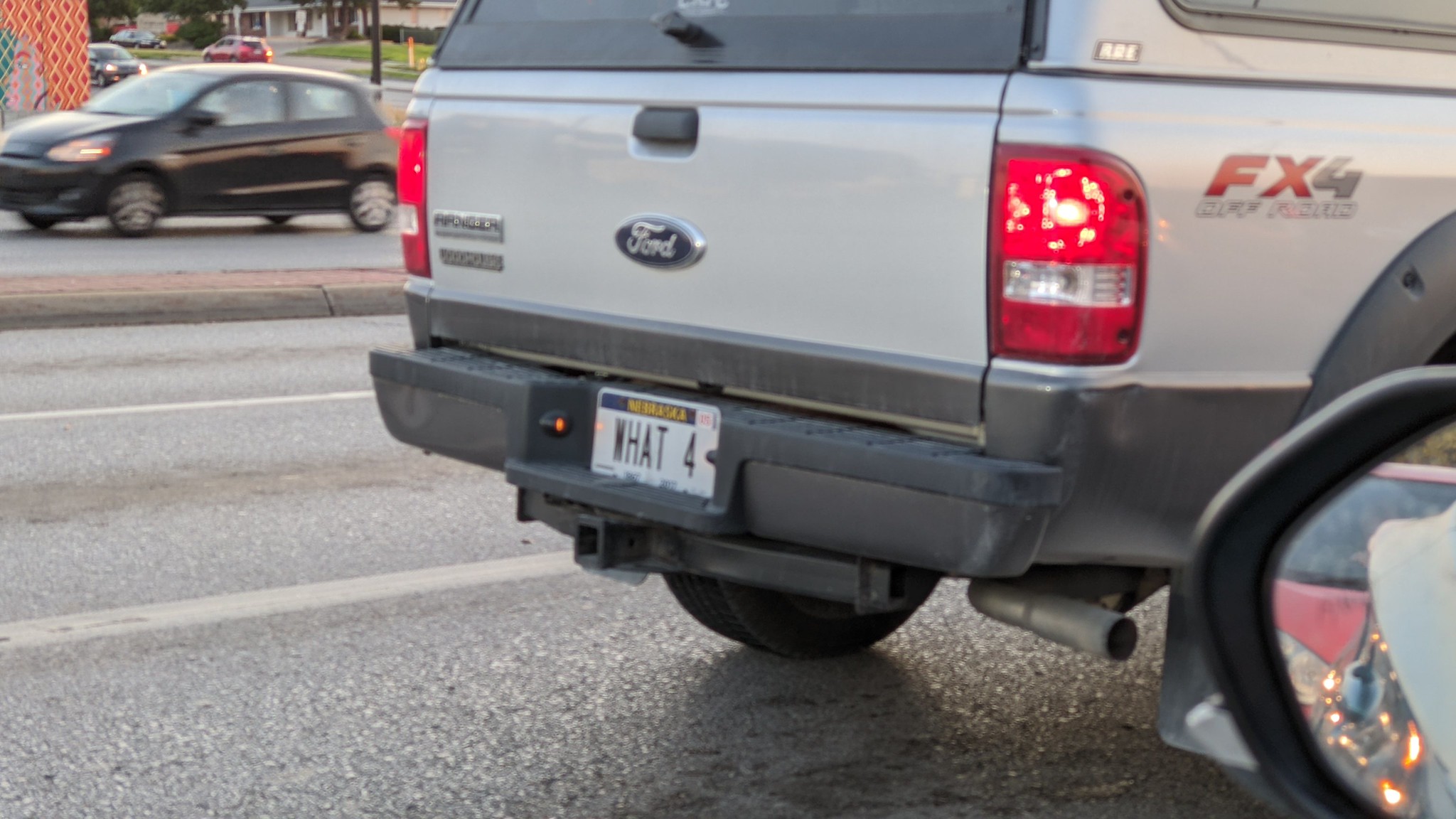This photograph, taken from inside a car, captures a detailed outdoor scene framed by a rearview mirror visible at the bottom right, with gray trim and a slight glimpse of a side mirror reflecting a red vehicle. The interior setting is confirmed by the close proximity and angle from which the image is taken. Dominating the center of the frame is a gray Ford FX4 truck featuring a black bumper, black wheel wells, and black trim around the windows. The truck's license plate is white with a blue banner and red lettering, though the state name is somewhat blurry, possibly Minnesota, Michigan, or Nebraska. The clear text on the plate reads "WAT4." The image also shows a roadway running through about two-thirds of the picture, separated by a concrete barrier and white lane markings. On the far road in the upper left corner, a black car is traveling from left to right. The truck appears stationary, likely stopped at a stoplight, indicated by visible brake lights and the context provided by the scene.